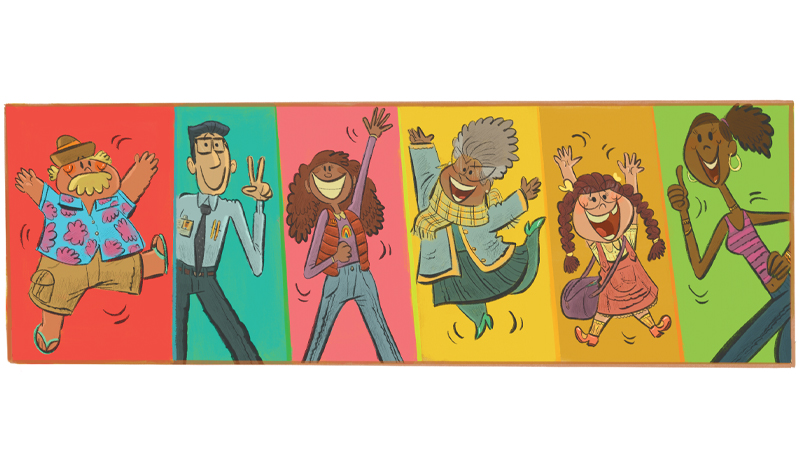This is a horizontally oriented, rectangular banner measuring approximately 3 inches high by 9 inches wide. The banner is divided into six sections, each featuring a cartoon illustration of a different character with a colorful background that changes from one panel to the next, moving left to right in the following order: red, turquoise, pink, yellow, gold, and green. 

In the first section with the red background, there is a larger man with a yellow blonde mustache and a little round brown hat. He is wearing a blue button-up shirt adorned with purple flowers, khaki cargo shorts, and blue sandals and appears to be flailing cheerfully with rosy cheeks. 

The second section has a turquoise background and features a white man in business attire consisting of a blue button-down shirt, tie, and gray slacks. He has glasses, an ID badge, and is throwing up a peace sign with a big smile on his face. 

In the third section, set against a pink background, is a dark-skinned girl with long, curly brown hair. She is wearing an orange puffy vest over a purple long-sleeved shirt, blue jeans, and has a huge smile while waving her hand exuberantly.

The fourth image on a yellow background features an elderly black woman with gray puffy hair. She is dressed in a plaid green, yellow, and black scarf, a long blue jacket, a teal skirt, teal stockings, and green high heels. She is jumping with excitement.

In the fifth section, with a gold background, there is a small Caucasian girl with long brown pigtails. She is dressed in a reddish-orange overall-style dress with a yellow shirt underneath. She is waving both of her hands in the air energetically, and is smiling widely, revealing a missing tooth. She also carries a purple satchel over her shoulder.

The last section has a green background and depicts a black woman wearing a pink and purple striped tank top. Her hair is tied back in a ponytail, she has hoop earrings, and blue jeans. She has one hand on her hip and the other hand giving a cheerful thumbs-up.

Every character in this lively banner is depicted with a joyful expression, adding to the vibrant and dynamic feel of the artwork.